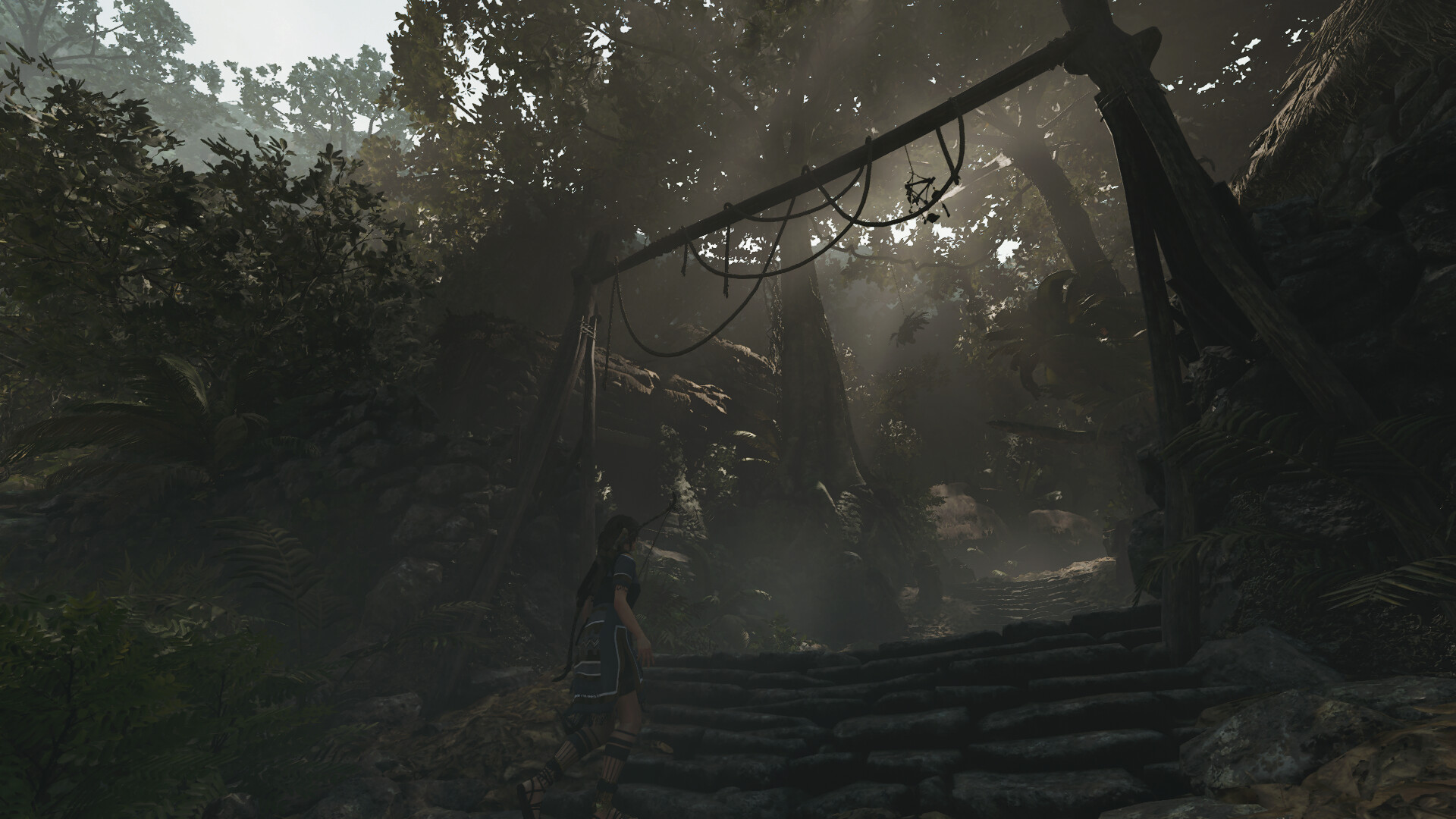The image appears to be a screenshot from a video game, depicting a dark and mysterious forest setting. There is a stone staircase in the lower right corner, leading upward into the dense trees bathed in a faint fog. This staircase is flanked by tall poles with ropes draping from a horizontal pole positioned diagonally above. Walking up the steps is a woman with long hair, likely an archer, as indicated by the bow and arrows she carries on her left shoulder. She is adorned in a short-sleeved tunic and stockings or long socks, paired with sandals. The character faces away from the viewer, heading towards a wooden archway that further enhances the entrance to the forest. The entire scene evokes the adventurous ambiance characteristic of a game like "Tomb Raider."